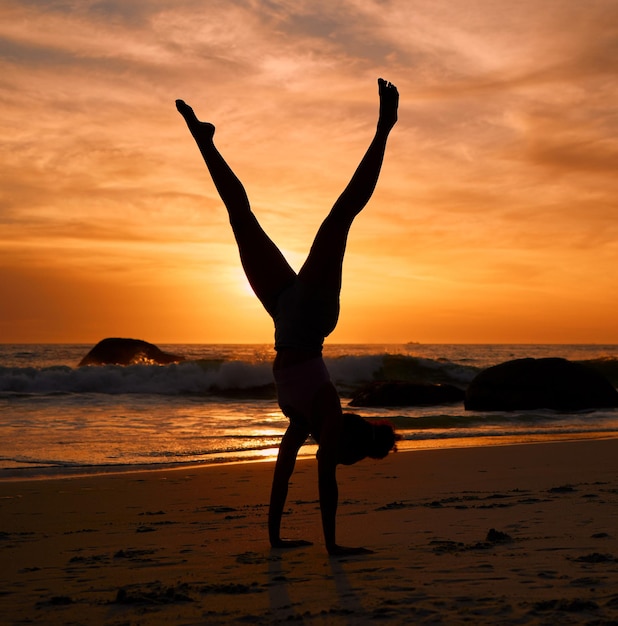In a photograph capturing the serene beauty of a beach at sunset, the sky is painted in rich hues of orange and yellow, gradually transitioning to a darker blue with wisps of white clouds towards the top. Below the skyline, the ocean's water glistens, with waves gently crashing against an extensive line of rocks that stretches from the left to the right of the image. In the foreground, the sandy beach is in low tide, clean and seemingly tropical. Dominating the scene is the dark silhouette of a woman performing a handstand on the sand. Her legs are extended upwards in a split, forming a V shape, and her bare feet point towards the sky. Her head, with hair tied up in a bun, is turned to the right, looking down at the sand beneath her, marked by numerous handprints. The glowing sun behind her sits low on the horizon, enhancing the dramatic contrast of the image.